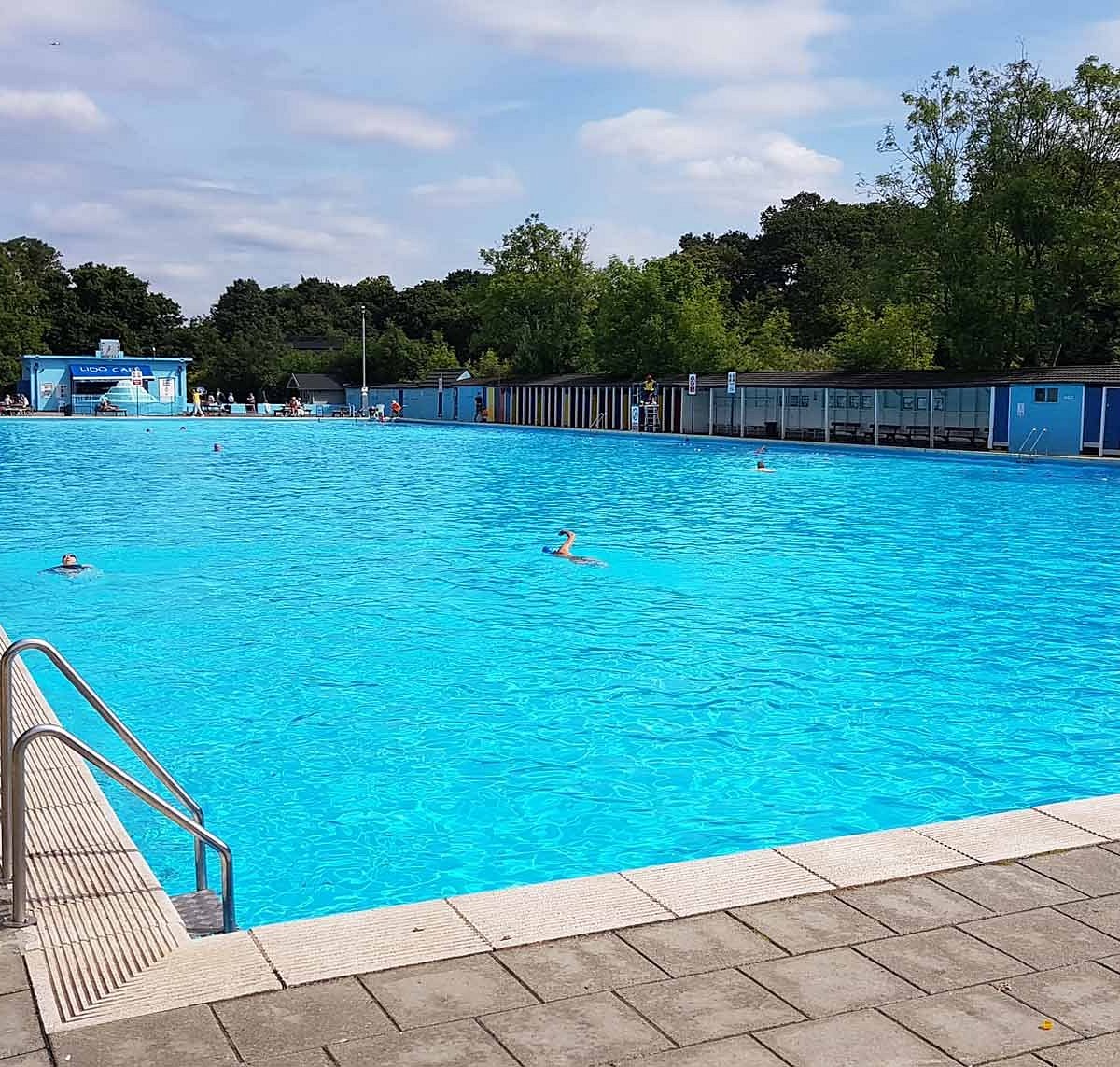The photo captures a beautiful and expansive public pool with vivid aqua blue water, enveloped by a gray-bricked walkway that transitions to lighter bricks bordering the pool. A silver metal staircase, located in the bottom left corner of the image, provides access into the inviting waters. On the far side of the pool, a blue building—likely a small snack stand or cafe—adorned with a sign that reads "Lido Cafe" stands adjacent to a fence that stretches across the right side and middle of the picture. In front of the snack stand, a colorful umbrella adds to the lively atmosphere. The pool itself hosts a few swimmers; some individuals' heads peak above the surface while others swim or float more visibly. Skating the perimeter, the scene is framed with lush green trees under a light blue sky filled with clouds, providing a picturesque backdrop. Scattered about, signs are visible across the pool area, though they remain unreadable from the viewer’s position. The overall ambiance captures a serene and welcoming environment for outdoor leisure.